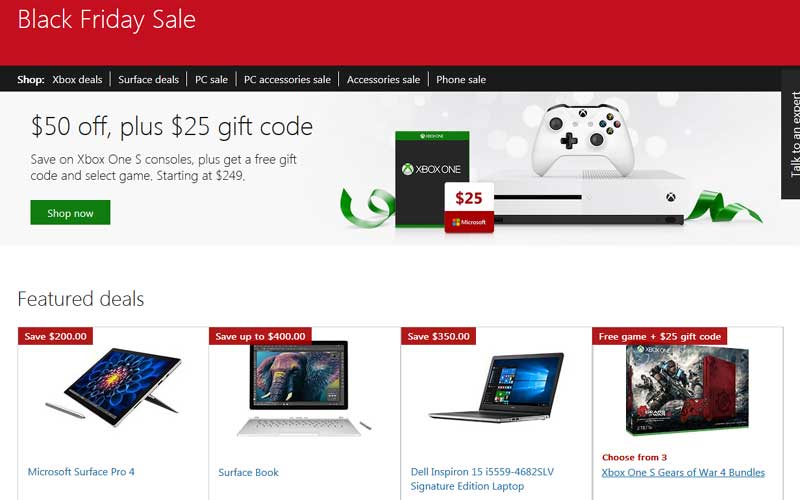Screenshot of a Black Friday Sale from an Electronics Retailer

The image captures a vibrant Black Friday sale advertisement from an electronics retailer's website. At the top, a prominent red banner stretches across the screen with the text "Black Friday Sale" written in bold white letters. Just below this, a black navigation bar offers various shopping categories including Xbox Deals, Surface Deals, PC Sale, PC Accessories Sale, Accessories Sale, and Phone Sale, ensuring a comprehensive, user-friendly experience.

The central portion of the screen features a detailed promotion for Xbox One S consoles. A large section of the screen, with a white background, highlights a special offer: "$50 off plus $25 gift code. Save on Xbox One S consoles. Plus get a free gift code and select game starting at $249," accompanied by a green 'Shop Now' button. To the right of this text, a vivid image displays an Xbox One S console with a matching controller, an Xbox One card, and a $25 Microsoft gift card, all set against a backdrop adorned with a green ribbon for added festivity.

On the right-hand side, a black box labeled "Talk to an Expert" offers additional customer support options, ensuring shoppers can get assistance with their purchases.

Below the featured Xbox One S deal, the screen showcases four additional remarkable offers:
1. Save $200 on a Microsoft Surface Pro 4.
2. Save up to $400 on a Surface Book.
3. Save $350 on a Dell Inspiron 15 i5559-4682SLV Signature Edition Laptop.
4. Free game plus $25 gift code: Choose from three Xbox One S Gears of War 4 bundles.

Each deal is accompanied by a corresponding image, further enticing potential buyers with visual depictions of the products.

The overall layout and design capture the essence of high-stakes Black Friday shopping, blending compelling offers with efficient navigation and attractive visuals.